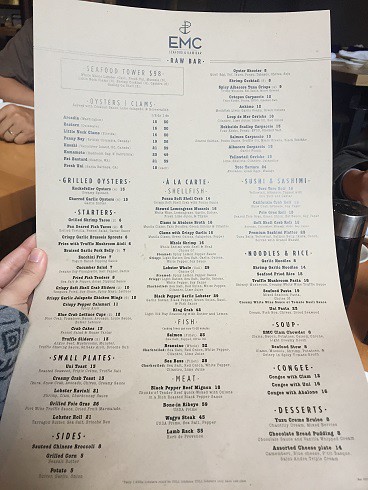This detailed image caption describes a bustling scene at a seafood restaurant.

"A close-up shot of a long, rectangular, tan-colored menu with blue and black text, held in a white hand adorned in a gray and blue sweater. At the top of the menu, 'EMC Seafood & Raw Bar' is prominently displayed. The menu comprises a variety of sections, including 'Seafood Tower,' 'Oysters and Clams,' 'Grilled Oysters,' 'Starters,' 'Small Plates,' 'Sides,' 'À la Carte,' 'Shellfish,' 'Fish,' 'Meat,' 'Sushi and Sashimi,' 'Noodles and Rice,' 'Soup,' 'Congee,' and 'Desserts.'

In the background, a lively restaurant scene unfolds with several tables occupied by patrons. Directly behind the menu holder, a white man wearing a wedding ring is visible at another table. Additional tables can be seen, some with diners and others empty, contributing to the vibrant and social atmosphere. The rich array of seafood options, including shrimp cocktails and raw fish, hints at the restaurant's specialty. The environment suggests a popular dining location characterized by a broad selection of fresh seafood dishes."